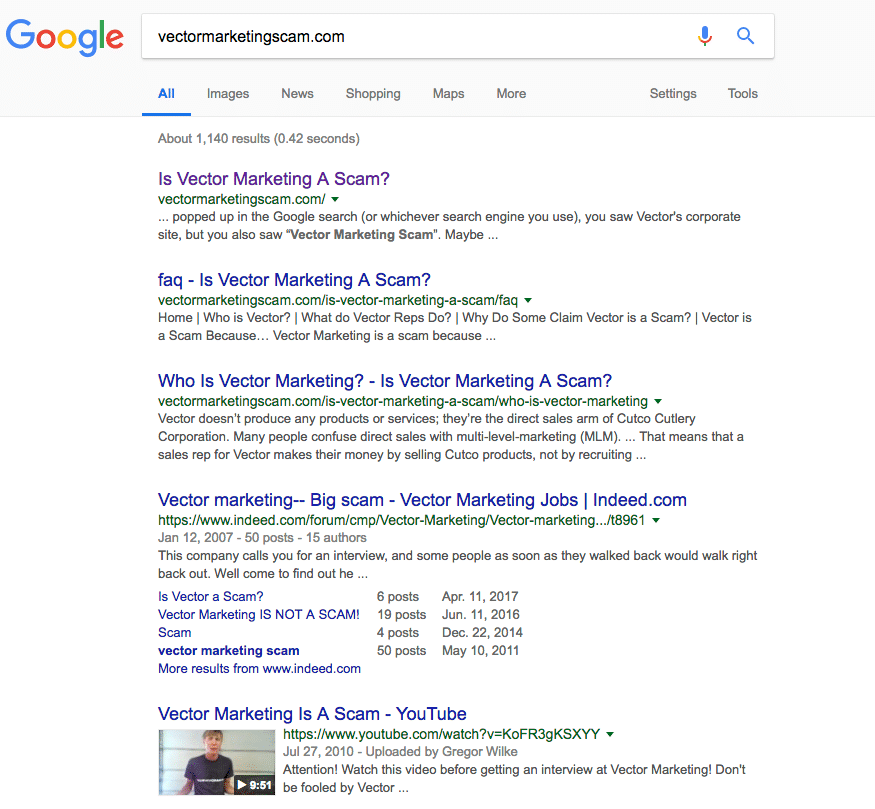An image depicts the Google search results page for the query "VictorMarketingScam.com". At the top of the page, the iconic Google logo is displayed in its vibrant rainbow colors. Below the logo, the search query is entered into the search box, and beneath this are the standard navigation options: All, Images, News, Shopping, Maps, More, Settings, and Tools.

The search yields approximately 1,140 results in a swift 0.42 seconds. The top results prominently tackle the inquiry regarding the legitimacy of Vector Marketing, with highlighted titles such as "Is Vector Marketing a Scam?" in dark blue text. One of the results is a frequently asked question, "Is Vector Marketing a Scam?", also in dark blue letters. Another key result provides an explanation on "Who is Vector Marketing?" Additionally, the fourth major result, "Vector Marketing, Big Scam, Vector Marketing Jobs," links to Indeed.com. 

The search results consistently question the credibility of Vector Marketing, offering detailed responses to queries like "Is Vector Marketing a Scam?". The corporate site for Vector is mentioned, as well as alternative results explicitly labeled as scams, reinforcing the theme of scrutiny surrounding Vector Marketing within the search results.